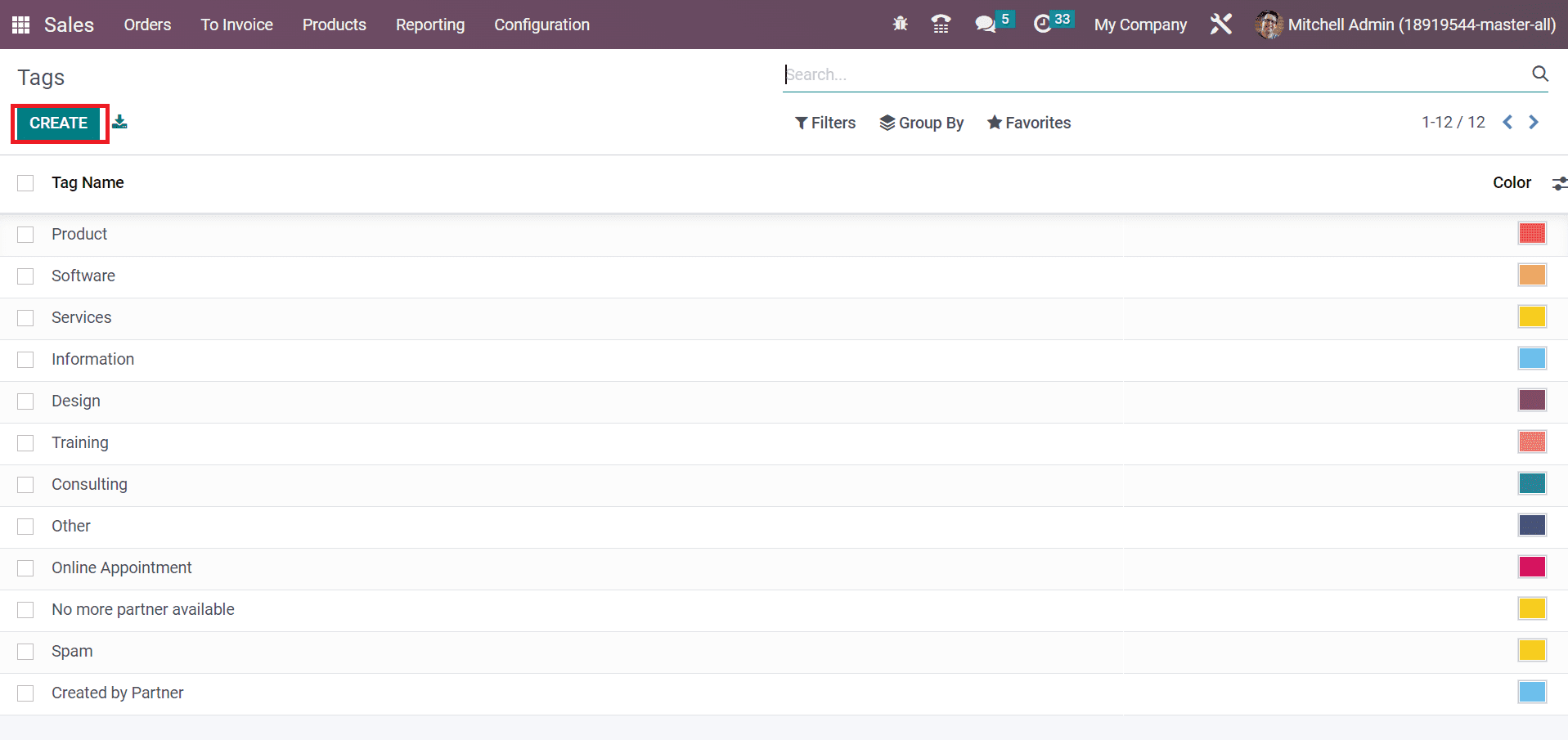This screenshot of a web page features a detailed navigation banner across the top, colored in dark brown with white text. From left to right, the banner includes the following menu items: "Sales," "Orders," "To Invoice," "Products," "Reporting," and "Configuration." Next to these text items are icons including a beetle and a phone with buttons. 

To the right of these icons is a message notification icon showing the number 5 in a square, followed by a clock icon with the number 33 in a green square, indicating notifications or tasks pending review. The company name, "My Company," is prominently displayed next. 

On the far right, there is a wrench and pencil icon, commonly used for editing or settings, followed by a circular profile photo of a man with dark hair, fair skin, and glasses. The text next to the photo reads: "Mitchell Admin 189-19544 Master All," signifying the user's name, identifier, and role or access level.